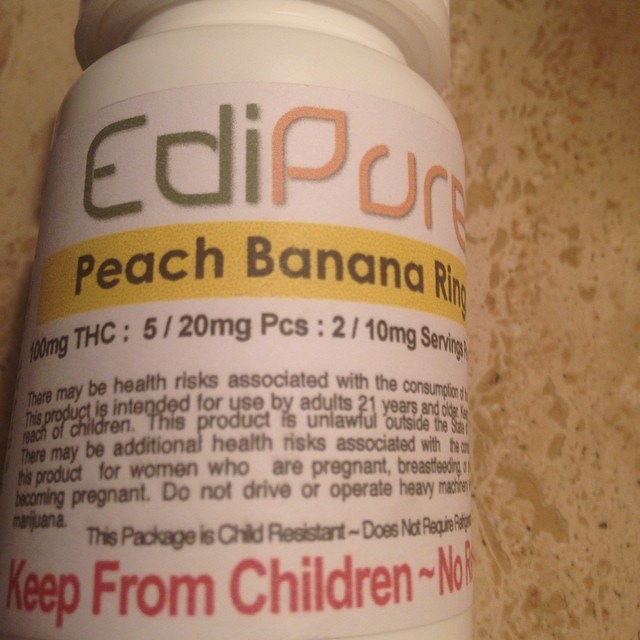The image depicts a close-up of a white, childproof pill bottle labeled "EdiPure." The bottle features a prominent yellow banner on the front displaying the flavor "Peach Banana Ring." The label details the product's THC content as 100 milligrams in total, divided into servings of two 10-milligram pieces, with each serving consisting of five 20-milligram pieces. The information also includes a clear health warning, advising the product is for adult use only (21 years and older), and to keep it out of the reach of children. Additional text on the bottle emphasizes that it is child-resistant and reinforces potential health risks associated with the consumption of this THC medication. The bottle is placed on a tan, marbled surface, enhancing the focus on the detailed labeling and health precautions.